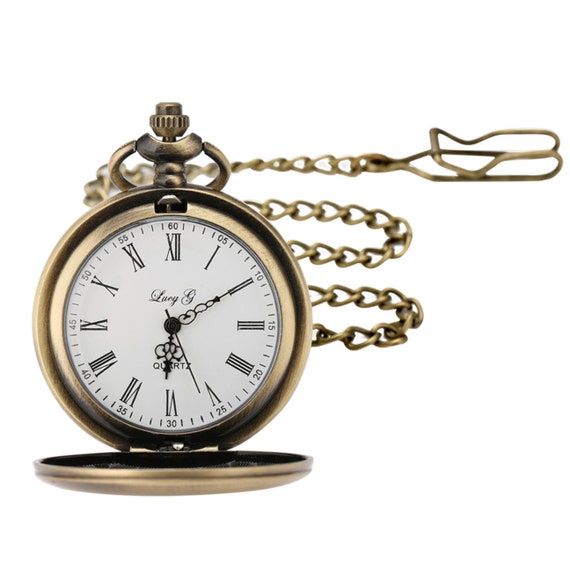This close-up image showcases a vintage pocket watch with exquisite details. The watch face is pristine white, encased in a sophisticated brushed silver metal that boasts a subtle matte finish, free from any shininess. Classic black Roman numerals adorn the watch face, providing a timeless elegance, while the black hands, including a slender second hand, add a touch of refinement with their intricate thin line designs. The time displayed is 6:10. The watch is in an open position, revealing the edge of its cover just below. At the top of the watch, the winder is prominently positioned. Lying behind the watch is a metal hook, part of an ornate chain. This chain emerges from the right center, looping back behind the watch and continuing its intricate pattern, eventually leading to another hook at the end. The ensemble captures the charm of a bygone era with meticulous attention to detail.